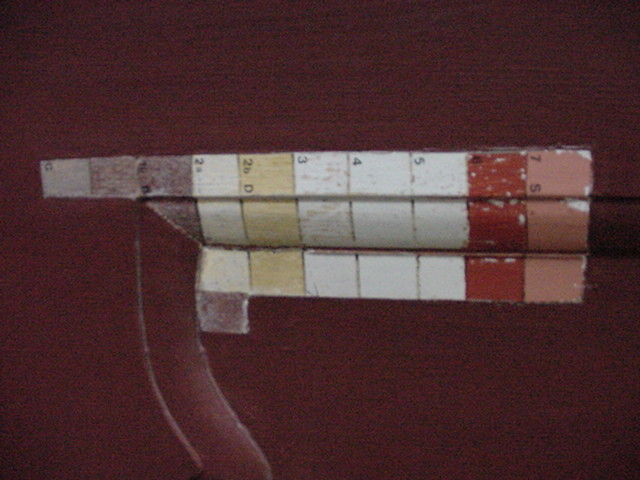In the image, set against a black background, there is an arrangement of one-inch square boxes, each marked with different numbers and letters: 7, 6, 5, 4, 3, 2B, and 2A. These boxes, which vary in color—including shades of red, salmon, white, off-white, yellow, black, and gray—are arranged in a pattern that vaguely resembles the shape of a gun. Specifically, the collective formation suggests the outline of a gun, with what seems to be a handle or magazine protruding downward. This handle-like feature transitions from the body and curves slightly, evocative of the long magazine seen on some submachine guns. Though the image might initially appear abstract or incomplete, it conjures the distinct impression of a firearm, potentially in an untextured or preliminary design phase.